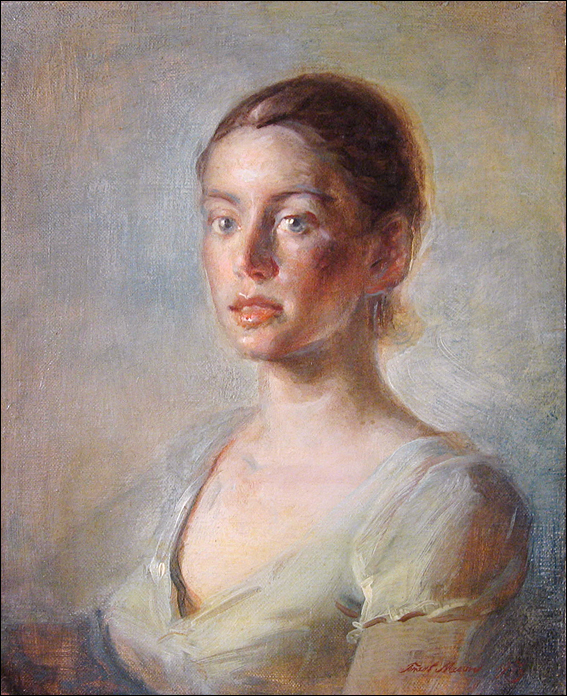This oil painting depicts a young Caucasian woman, portrayed in a formal, Victorian-era style. The close-up perspective reveals her head, shoulders, and bust. She has light skin, glossy peach-colored lips slightly parted to show her front teeth, and blue or green eyes. Her hair, which could be dark blonde, brown, or dark red, is swept away from her face and pulled into a bun at the back. The woman is dressed in a light-colored, silky-looking dress with a deep V-neck and puffed shoulders that taper at her upper arms. The color of the dress is ambiguous, with hints of off-white, gray, light yellow, or tan. She is depicted without any jewelry other than potential silver earrings, though this detail is contested. The background blends smoky grays, yellows, and blues, adding an atmospheric touch to the portrait. The artist's signature appears in red cursive in the lower right-hand corner of the artwork.